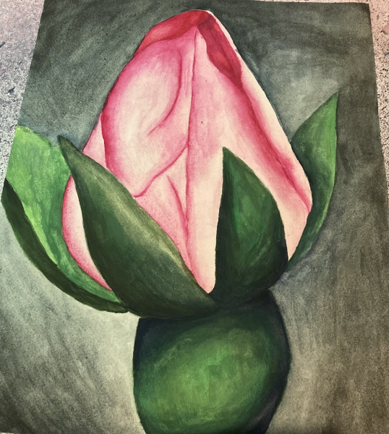This detailed piece of color artwork, rendered on a canvas-like material, features a delicate rosebud poised to bloom. The rosebud, primarily pink with accents of darker red, is enveloped by four green petals that are beginning to open, revealing the flower. The petals are elegantly positioned, with two in the front and one on each side, creating a natural framing for the rosebud. Beneath the petals, the bulb of the flower is rounded and painted in various shades of green, from hunter green to lighter and yellowish tones, adding depth and realism to the piece.

The background of the artwork is filled with textured black shading, interspersed with lighter tones and gray scribbles, particularly around the rosebud, to highlight its delicate details. This entire composition, devoid of any writing, people, animals, buildings, or signs, is situated on a speckled marble-like gray surface, emphasizing the focus on the budding flower.